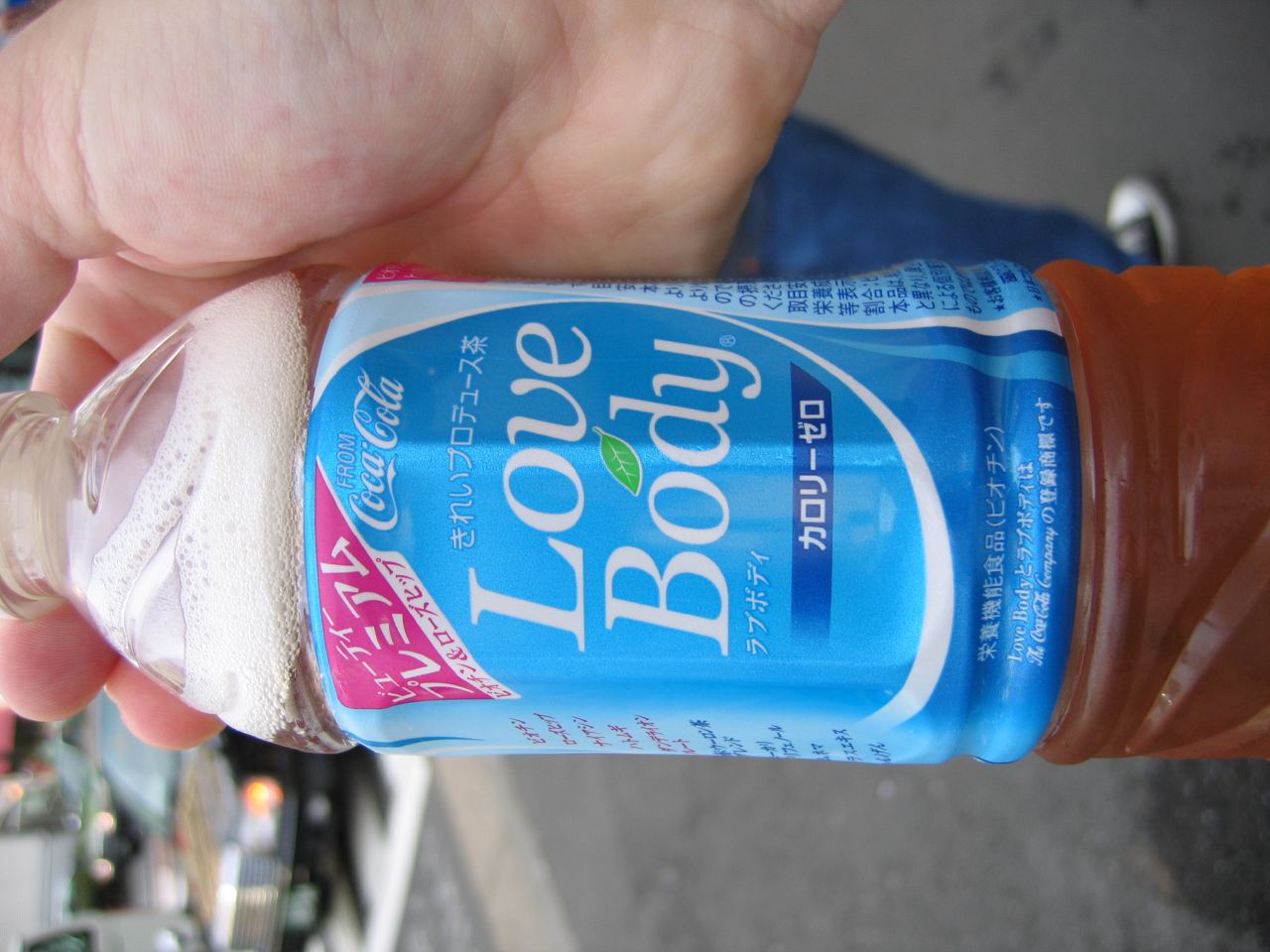In this outdoor photograph, a pale-skinned right hand grips a clear, translucent plastic bottle around the neck. The beverage inside is a light amber-brown color with a bit of foam at the top, suggesting it has been recently shaken. The blue label on the bottle features a variety of characters, likely Japanese or Chinese, which are unreadable to the viewers. However, in white letters, it prominently displays the words "love body," separated by a small green leaf image. Above this text, it reads "from Coca-Cola" in white font. There's a hot pink triangle toward the top left of the label with additional characters. The background reveals what appears to be a parking lot with tarmac, featuring several parked cars and a glimpse of a person's leg and foot dressed in blue jeans and black fabric Converse sneakers with white toes and laces.